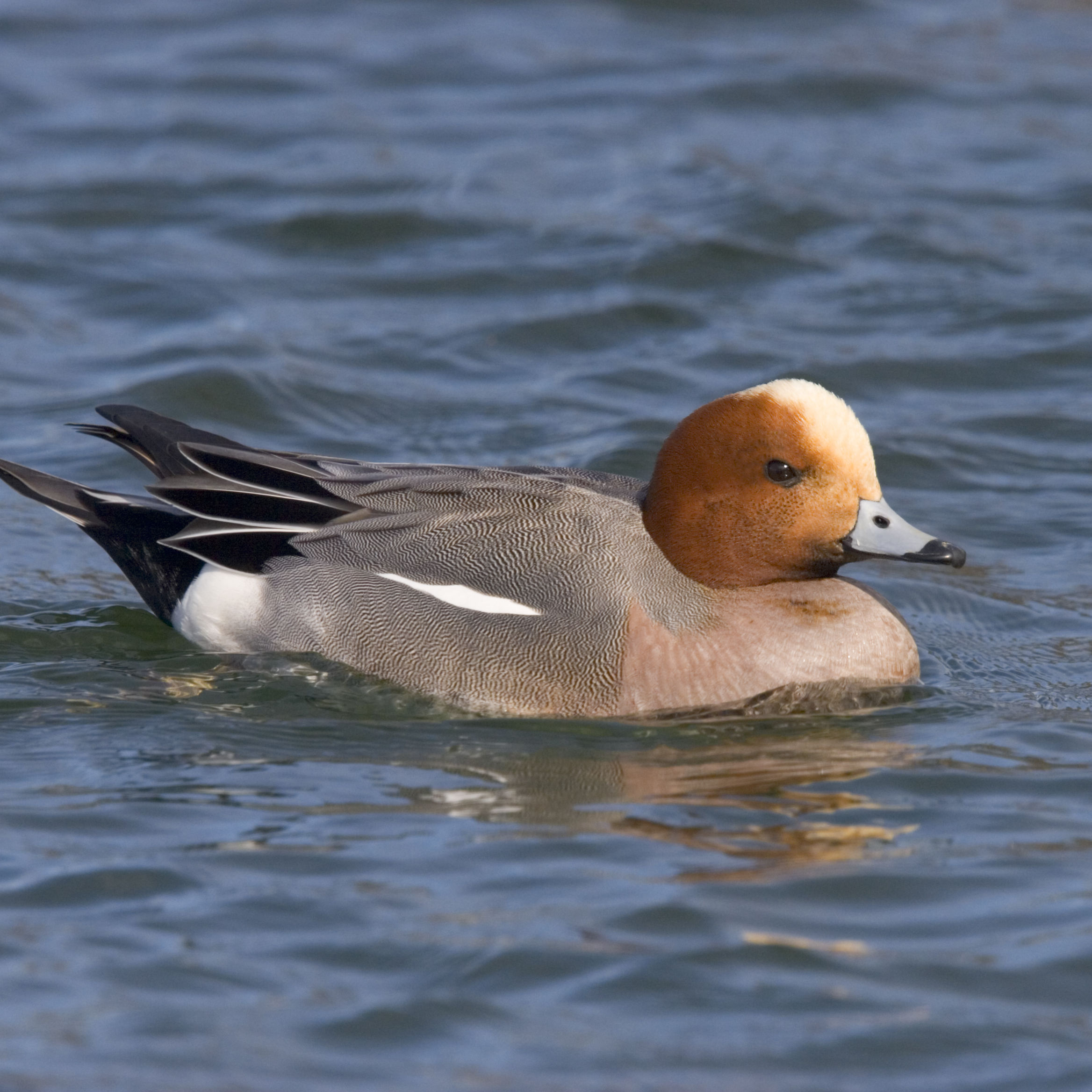This is a detailed photograph of a striking duck floating in a slightly wavy, grayish-blue body of water, situated in the middle of the rectangular image, which is slightly taller than it is wide. The duck features an orange-brown head adorned with a distinct white stripe running from its beak to the back of its head. Its beak is uniquely colored, with the front third being black, followed by a gray section that has a notable black dot resembling a nostril. The beak also has a curved tip. The duck's spherical black eye stands out against its orangish-brown head. It is facing to the right, exposing the right side of its body and head.

The duck's body begins with pinkish-white feathers at the front, transitioning to a section of white and black with alternating squiggly lines, resembling polka dots. Towards the rear, the feathers darken to black, accented with white outlines, culminating in a black tail contrasted by a white rump. The water around the duck is a blend of greenish-blue hues with visible ripples, adding a dynamic quality to the serene scene.